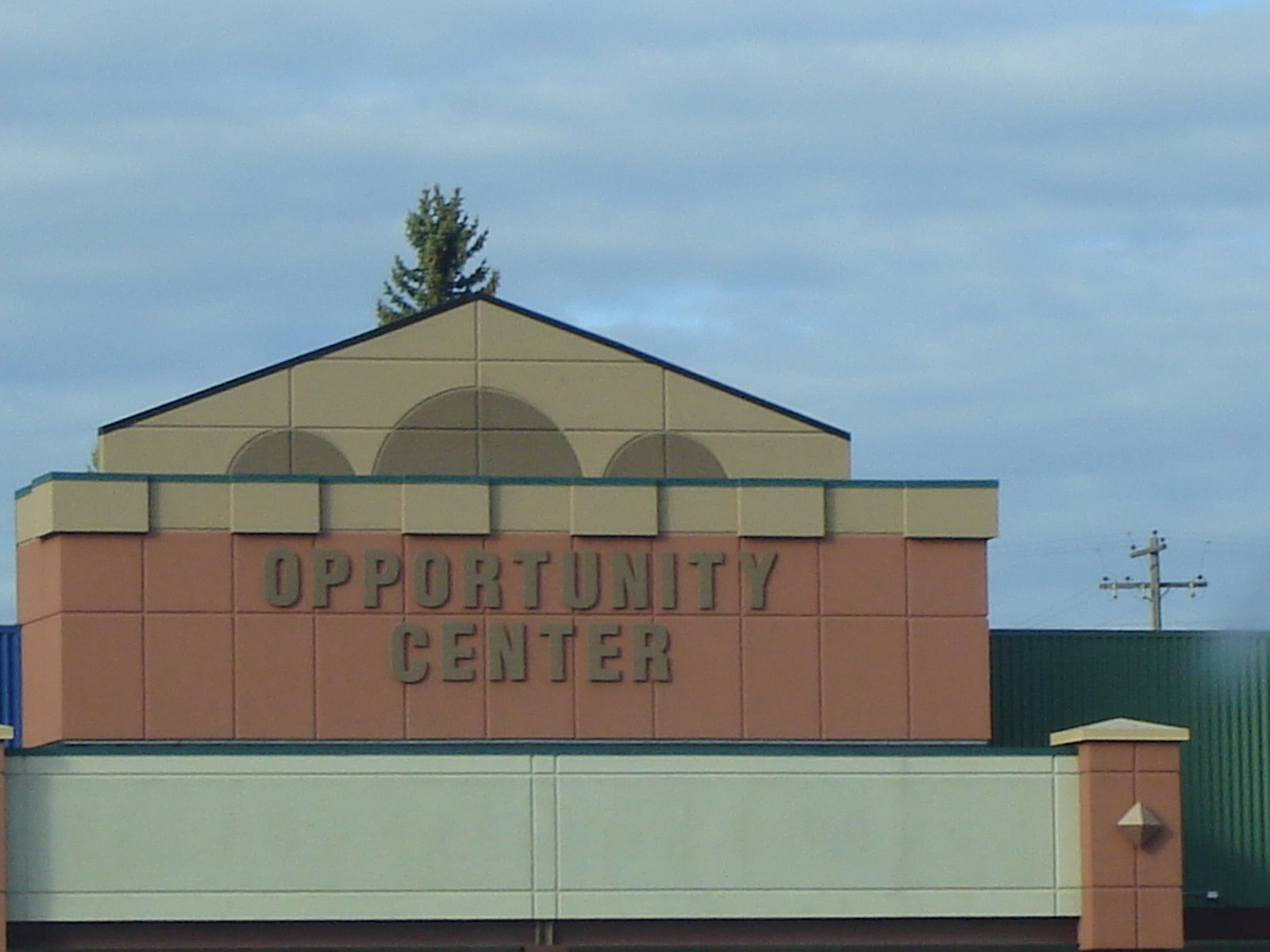A serene blue sky forms the backdrop of this vibrant urban scene. Dominating the background is a towering tree, its lush foliage adding a touch of nature to the environment. Nearby stands a tall electric pole, festooned with an intricate web of wires stretching across the frame. In the mid-ground, a substantial fence runs parallel to a large, multi-material building. The lower portion of the building features robust red bricks transitioning into lighter, concrete blocks as they rise. 

The structure's upper section is a light brown, boasting three darker brown arches that lend it a distinct architectural flair. Prominently displayed in brown letters across the edifice is the text "Opportunity Center." Adjacent to it, a contrasting black segment supports large white blocks with black bases. Finally, the scene is punctuated by a red element adorned with a central gold star, topped off with a light-colored peak, adding a sense of whimsy and detail to the urban landscape.